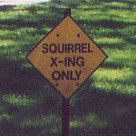This is a small, low-resolution image featuring a yellow, diamond-shaped sign with a black outline, mounted on a black pole. The sign prominently displays the text "SQUIRREL X-ING ONLY" in all capital letters. The background is mostly grass, varying in shades of green from very dark to bright, indicating areas of shade and sunlight, possibly from an unseen forest area above. The grass appears pixelated, adding to the low-resolution quality of the image. The grassy background undulates, suggesting a hill behind the sign, which covers the entirety of the image.